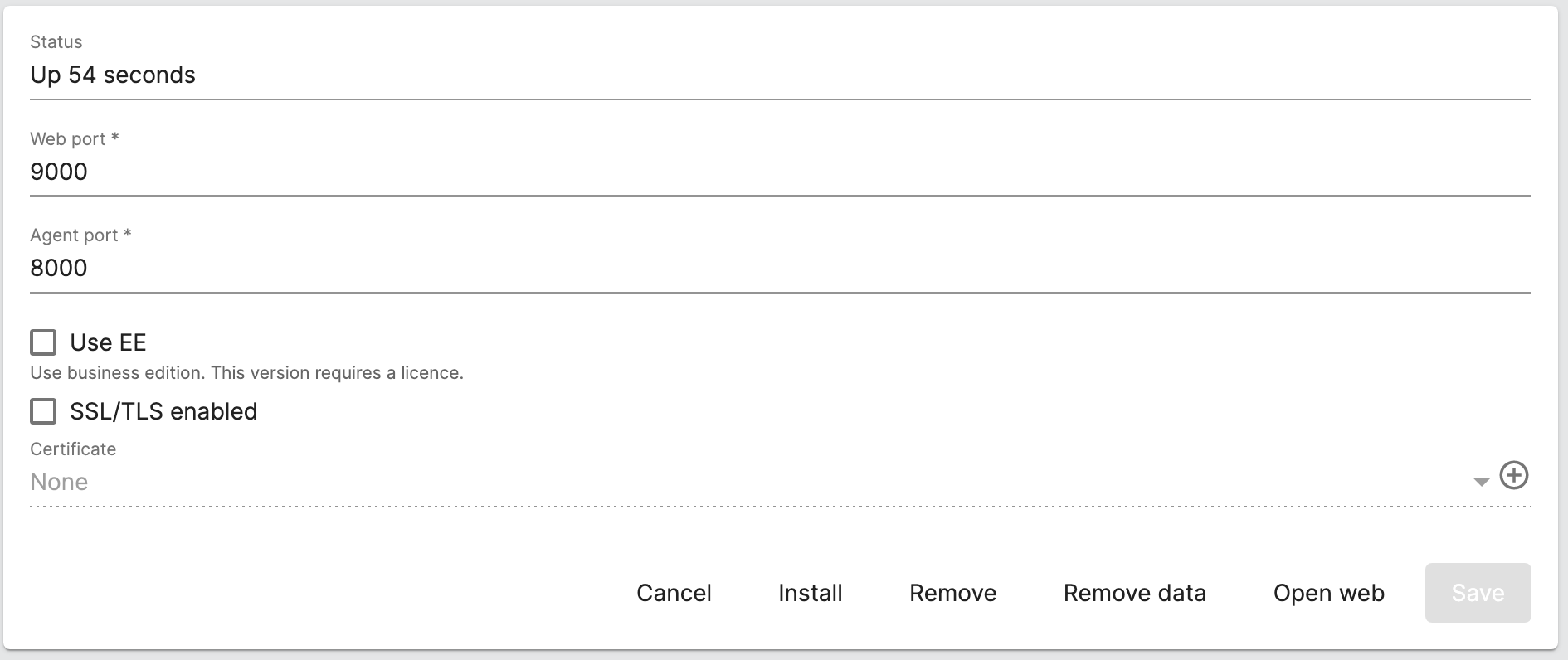**Image Description: Configuration Service Settings Interface**

The image depicts a settings interface for a configuration service, designed for quick and efficient setup. The key elements in the interface are as follows:

1. **Status Display**: The status is shown as "up to 54 seconds".

2. **Port Configuration**:
   - **Web Port**: Set to 9,000.
   - **Agent Port**: Set to 8,000.

3. **Configuration Options**:
   - **Use Business Edition**: A checkbox that requires a license; this box is not checked.
   - **SSL/TLS Enabled**: A checkbox indicating whether SSL/TLS is enabled; this box is not checked.

4. **Certificate Section**:
   - A drop-down menu for selecting a certificate is displayed just below the SSL/TLS checkbox and it is currently set to "None".

5. **Action Buttons**:
   - **Cancel**: To cancel the changes.
   - **Install**: To initiate the installation process.
   - **Remove**: To uninstall the service.
   - **Remove Data**: To delete associated data.
   - **Open Web**: To open the web interface.
   - **Save**: Currently inactive, indicating no changes have been made for saving.

The interface has a clean and straightforward design, emphasizing ease of use for configuring various service settings such as ports and security features.